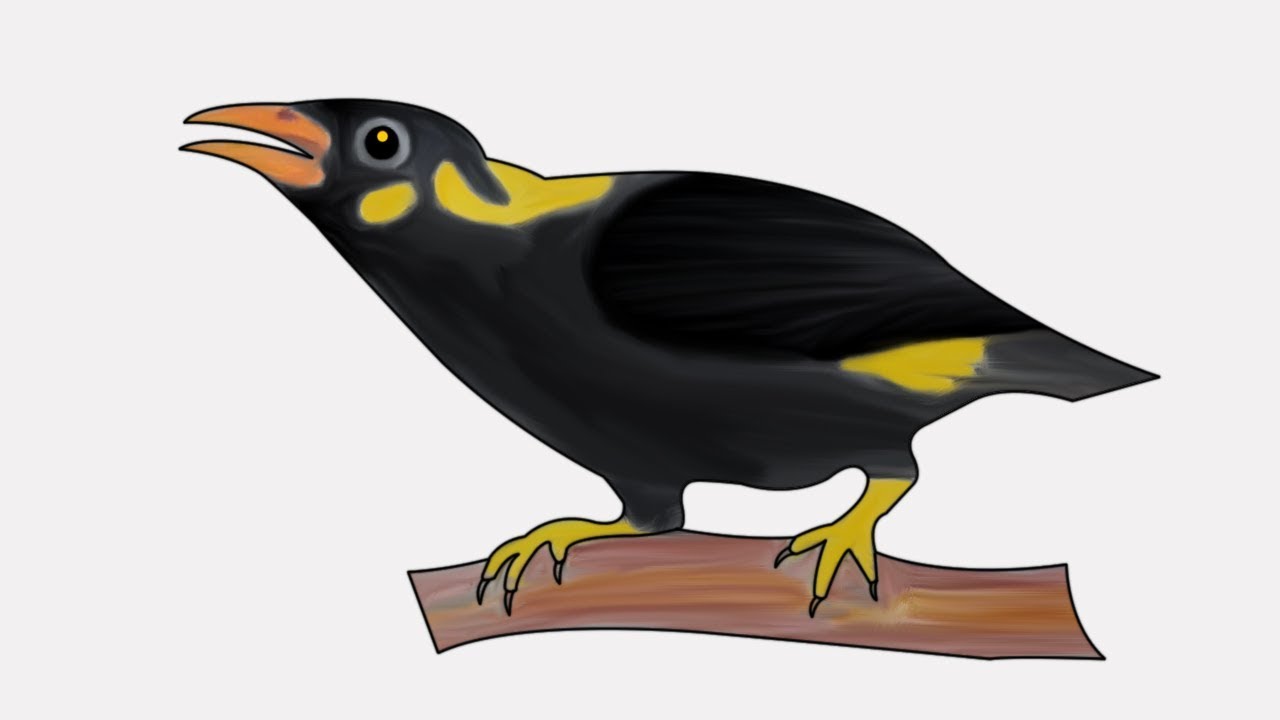The rectangular image, approximately six inches wide by three inches tall, features a detailed painting of a distinctive black bird with yellow accents perched on a stylized branch. The background is a light gray with a subtle lavender tinge, adding a soft contrast to the vivid colors of the bird and branch.

Central to the composition, the bird is depicted facing left, showcasing its striking orange beak, which is nearly the length of its head. The bird's eye is black with a yellow dot in the center, encircled by a lighter gray area. The plumage of the bird is predominantly black, but there are notable yellow markings: an oval patch under its eye, some yellow on its back, a small yellow part under its wing, and yellow legs and claws with three talons gripping the branch.

The branch itself is richly colored with stripes of different browns—dark brown, light brown, and reddish brown—and touches of bluish-gray. These shades give the branch a textured and stylized look that complements the overall color scheme of the artwork. 

Together, these elements create a visually appealing image with intricate details, vividly capturing the essence and beauty of the bird.